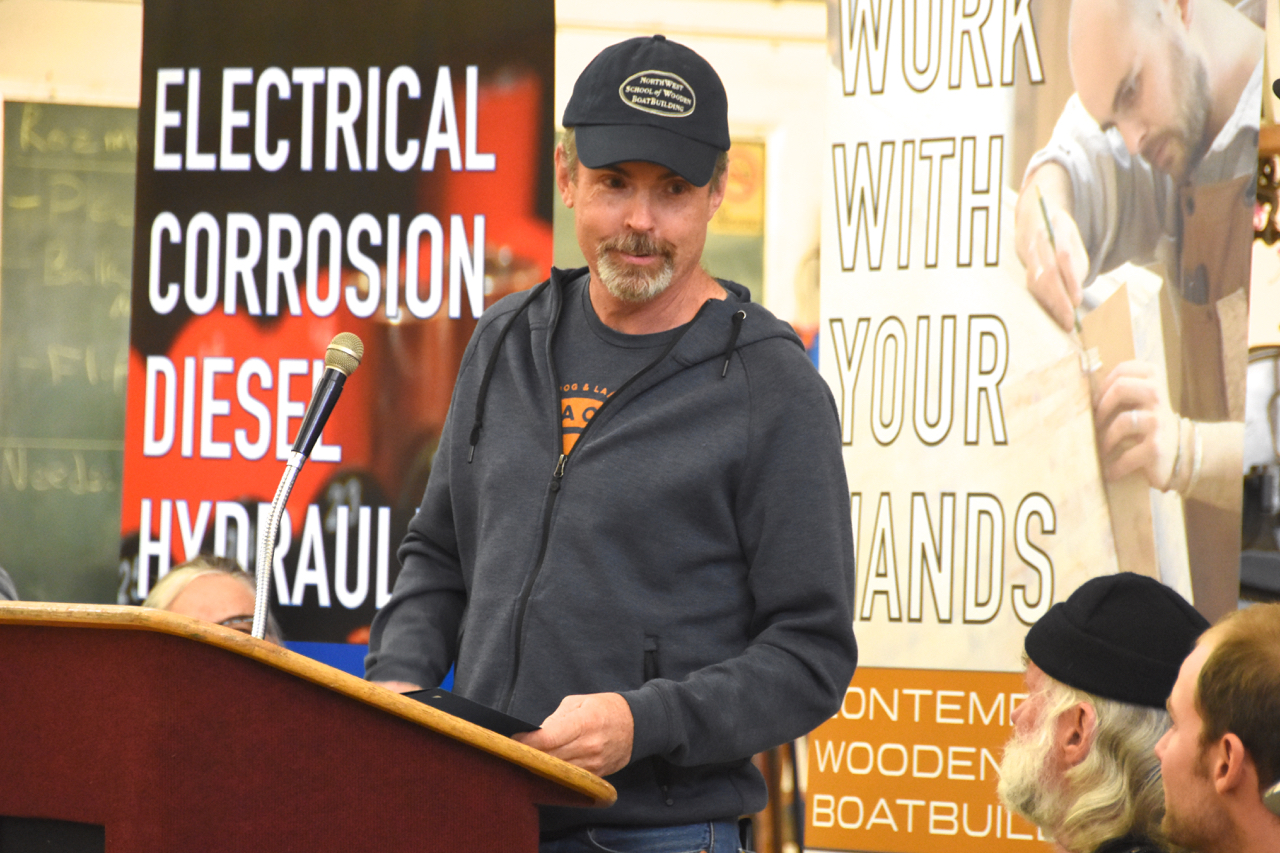This color photograph captures a moment at an educational event. At the center, a man stands at a two-toned wooden podium with a microphone protruding. He is dressed casually in a gray zip-up hoodie over a t-shirt, possibly paired with jeans, and a black baseball cap that reads "Northwest School of Wooden Boat Building." His gaze is directed to his left, seemingly engaged in answering a question posed by one of the onlookers. To his right, two men listen attentively: one with a white beard sporting a black knit cap, and the other looking up, engrossed in the speaker's response. Behind the main subject, two signs flank the scene. The sign on the left lists topics such as "electrical corrosion," "diesel," and "hydraulic," though partially obscured by the man. The sign on the right, set against a white background, encourages hands-on work with the text "work with your hands," accompanied by an image of a person crafting a wooden piece. The overall setting suggests a focus on practical skills and craftsmanship, possibly within a maritime or boat-building educational context.